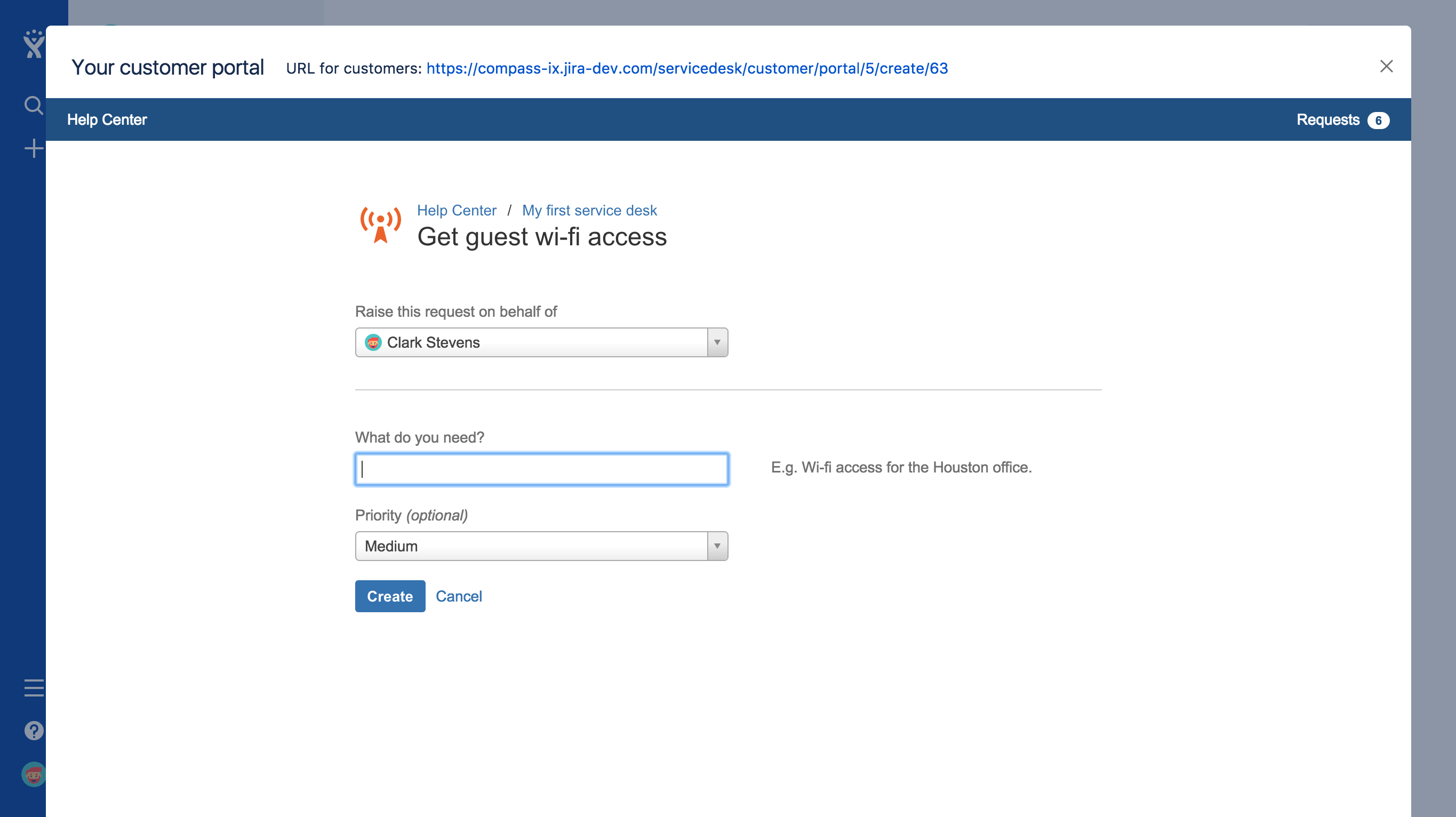The image displays various graphical elements arranged neatly within a structured layout:

1. **Left Column:**
   - A dark blue rectangle extends partially from the top.
   - Below it, a bluish-grey rectangle transitions into a slightly larger grey rectangle towards the bottom.

2. **Central Area:**
   - A white rectangle with the text "Your Customer Portal" on the left, followed by some illegible smaller text and a blue-colored website link.
   - A grey "X" is located on the right to clear or close the window.

3. **Middle Section:**
   - Another blue rectangle on the left labeled "Help Center."
   - Adjacent to this, a faint white oval with black text inside—content unclear.
   - The main visual features an orange-yellow triangle with a central dot. Surrounding this are two curved lines on either side, expanding outwards.
   - The title reads "Help Center - My First Service Desk" followed by the option "Get Guest WiFi Access."
   - Additional small text is too blurry to interpret.

4. **Lower Segment:**
   - A grey-outlined circle or a slightly rounded rectangle that features a blue dot with an orange circle in the middle. The text inside is too small to read.
   - Further down, a grey square with a downward arrow.
   - It is followed by more text boxes, each containing tiny, unreadable words.
   - There’s a blue-outlined box with a line within it, and more text boxes below, also filled with diminutive text.

5. **Bottom Section:**
   - Another grey-outlined box that reads "Medium."
   - Nearby, a grey square with a downward arrow.
   - Buttons labeled "Create" in a blue rectangle and "Cancel" in blue text are aligned to the right.

Overall, this layout appears to be an interface for a customer portal or help desk system, featuring navigational and form elements where the specifics are largely rendered in tiny, indistinct text.